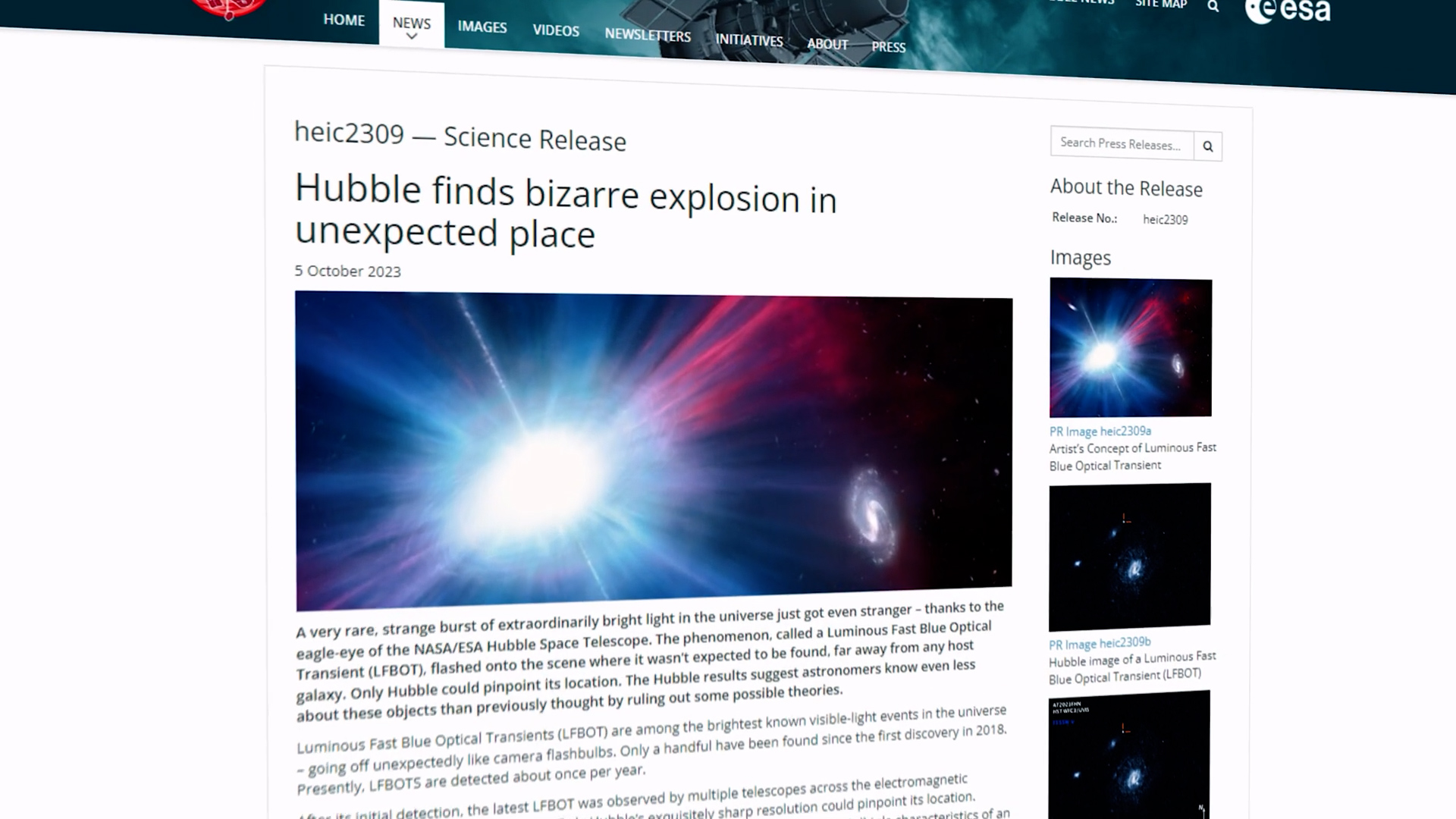This photo captures an angled view of a website, emphasizing its rightward tilt which leaves part of the screen cut off. The website's logo is not visible, but the bottom sections of the header can be seen, featuring categories such as Home, News, Images, Videos, Newsletters, Initiatives, About, and Press. The 'News' category is currently selected. 

The main content displayed is an article titled "Hubble Finds Bizarre Explosion in an Unexpected Place," with a heading that reads "HEIC 2309 Science Released". It is dated 5 October 2023, shown in small text to the left of a large rectangular image depicting a space explosion. The article's text continues below the image but is partially cut off, with the third paragraph truncated. 

To the right side of the screen, there's a panel titled "About the Release." This panel includes information such as the Release Number, followed by its corresponding number, and a section labeled "Images" which showcases three square thumbnail images with titles below each.